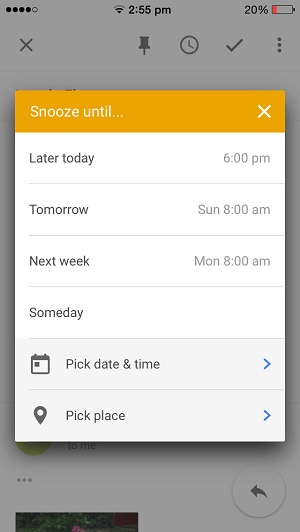The screenshot captures the clock settings interface. At the top of the screen, the current time is displayed as 2:55 PM. Below, within the clock settings, a yellow bar labeled "Snooze Until" presents various snooze options.

The options listed under "Snooze Until" include:
- Later Today, 6 PM
- Tomorrow, Sunday, 8 AM
- Next Week, Monday, 8 AM
- Someday, which appears blank.

Two additional icons and their functionalities are displayed below the snooze options:
- A calendar icon, which indicates "Pick Date and Time."
- A hot air balloon icon, labeled "Pick Place."

Both icons are highlighted with blue arrows on the right, suggesting they are interactive options. The entire interface is set against a clean white background, making the yellow bar and interactive elements stand out prominently.